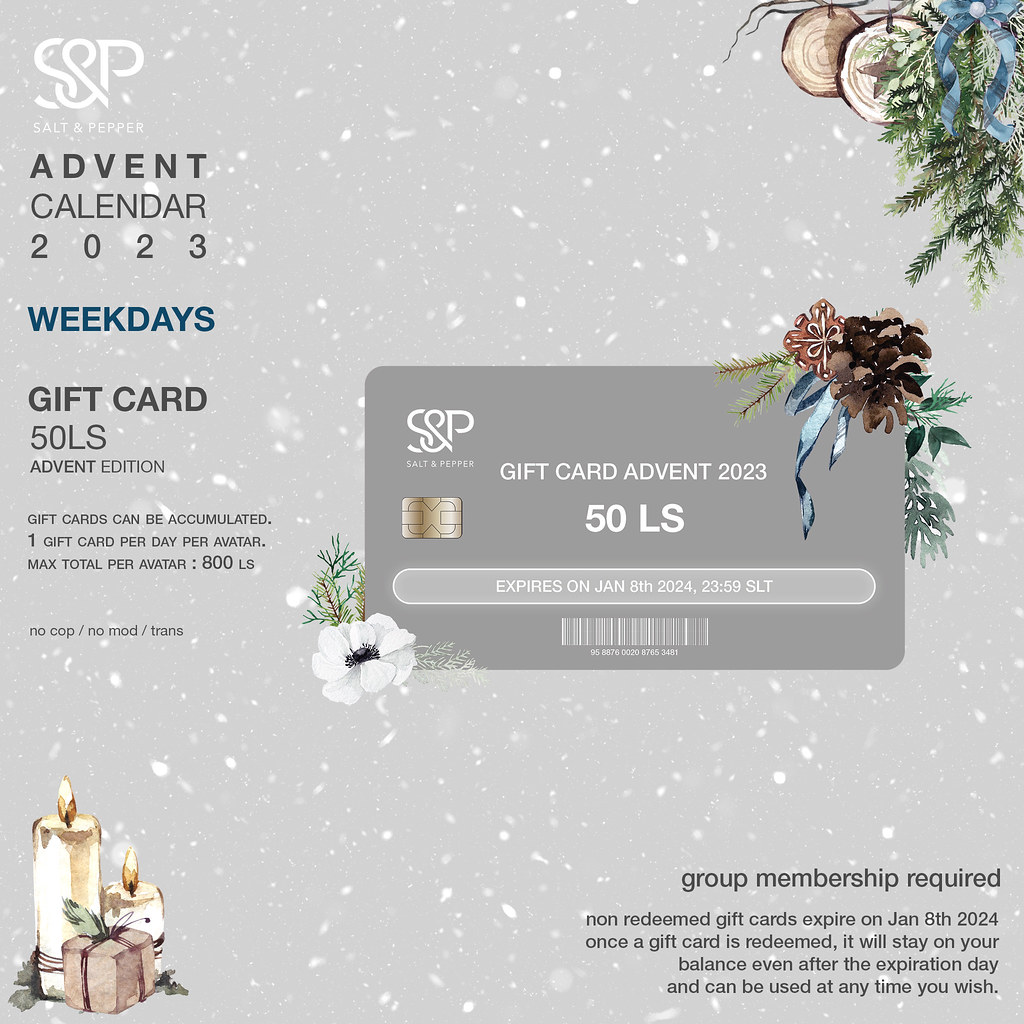The image is an advertisement for an S&P Salt-N-Pepper Advent Calendar 2023 Gift Card promotion, framed in a festive Christmas theme. The background is light gray with white snowflakes, creating a snowy effect. In the top left corner, the S&P logo appears with "Salt-N-Pepper" emblazoned underneath, followed by the text "Advent Calendar 2023" in bold black letters. Below that, in dark blue text, is the word "weekdays," and beneath it are the words "gift card" in bold black, along with the denomination "50 LS" and the label "Advent Edition."

In the center of the image is a gray gift card, decorated with a pine cone and green pine bough with a blue ribbon in the top right corner, and a white flower with a green branch emerging from the bottom left. The gift card reads "S&P Salt-N-Pepper Gift Card Advent 2023 50 LS," with an expiration date of January 8th, 2024, at 23:59 SLT, and a barcode at the bottom. To the bottom left of the image, there are two lit white candles and a wrapped beige package with a bow in front. In the bottom right corner, black text indicates "Group Membership Required" and notes the expiry details of the gift cards: non-redeemable cards expire on January 8th, 2024, but redeemed cards remain valid on the balance for use at any time.